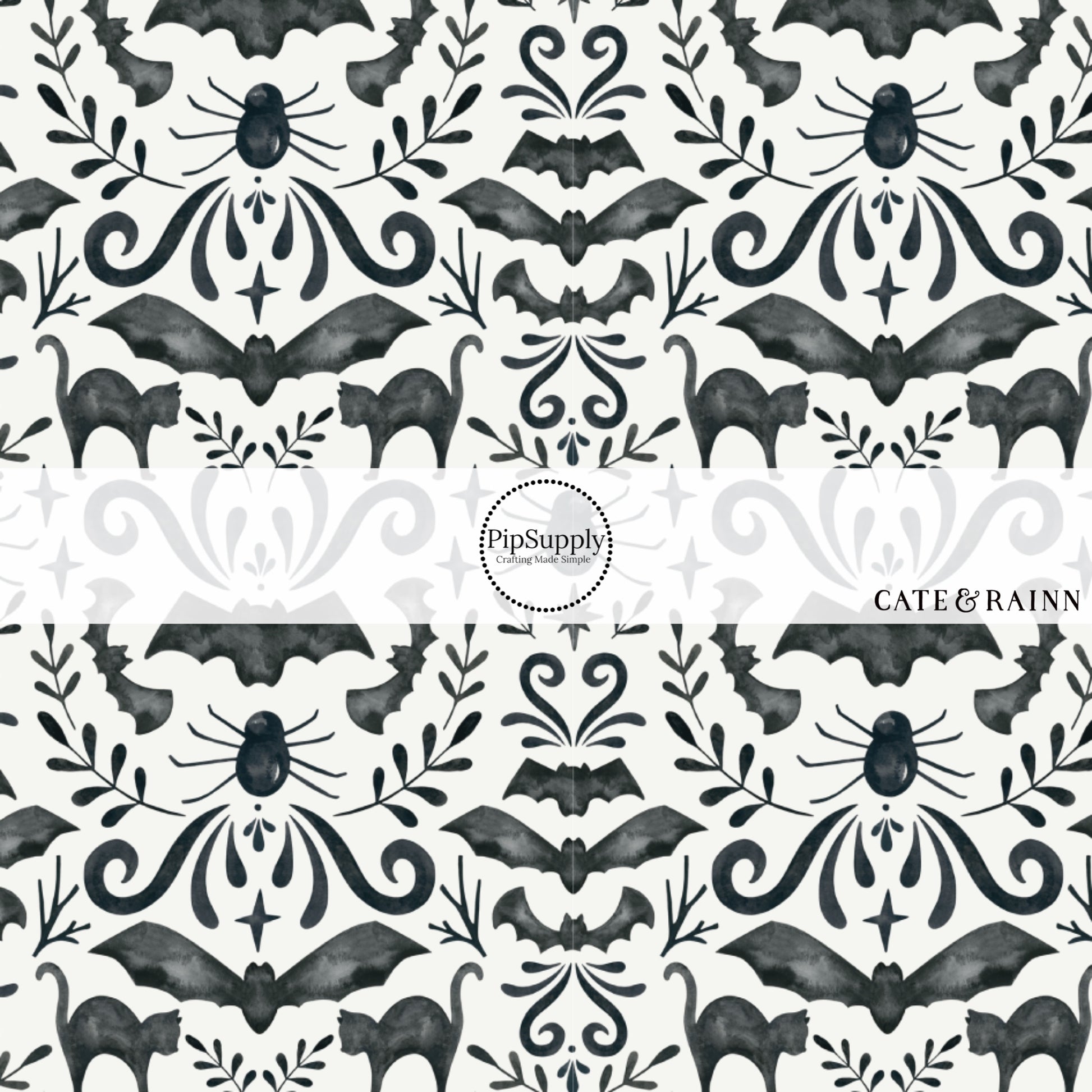The image depicts a seamless black and white patterned design, featuring Halloween-themed elements such as bats, black cats, spiders, and leaf-like decorations. In the center, there is a white label with black print. Within a circular arrangement in this label, it prominently reads "Pip Supply" along with the tagline "Crafting Made Simple." To the right of this circle, it displays "Kate & Rain" with "Rain" spelled with two 'N's. The repeating patterns suggest versatility, potentially making it suitable for use as wrapping paper or as a digital print for advertising purposes. The overall aesthetic hints at a spooky, yet stylish feel, aligning with a Halloween motif.